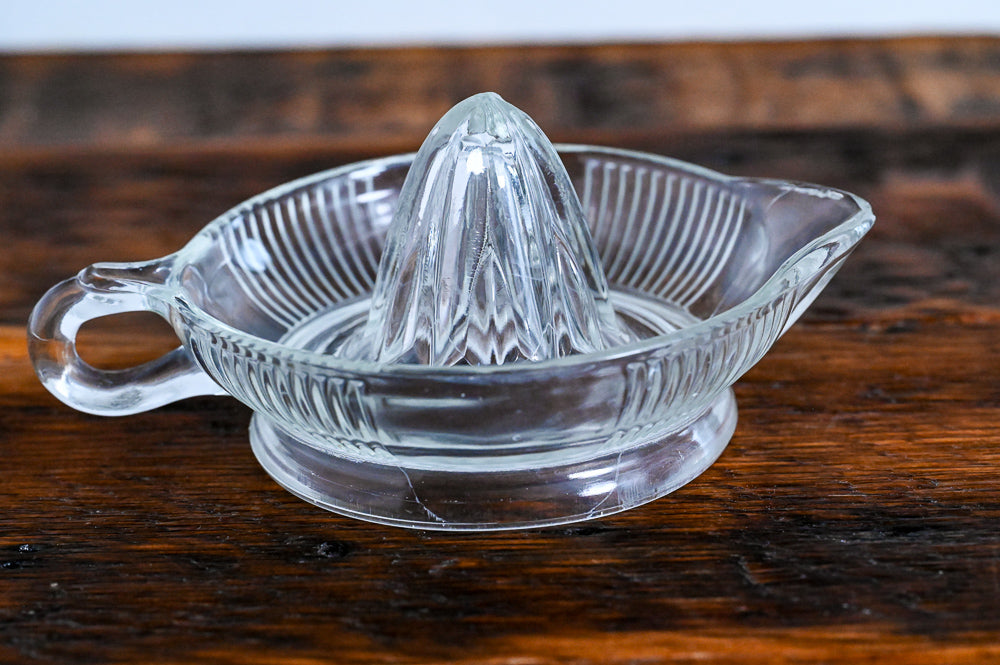The well-lit, clearly focused photograph captures a vintage glass citrus juicer situated on an antique, rustic wooden table. The table, occupying the background, features a matte finish with a rough texture, showcasing striated wood grains in a chestnut brown hue punctuated by darker brown patches resembling burn marks. The wood surface curves slightly upwards at the top of the image, maintaining its antique allure.

Dominating the composition is the glass citrus juicer, also known as a lemon reamer or orange squeezer. The juicer, reminiscent of Aladdin’s lamp in shape, comprises a shallow bowl with a spout on the right and a small loop handle on the left. The central feature of the juicer is a towering, cone-shaped projection used for extracting juice from halved citrus fruits. The glass vessel, adorned with four decorative ribbed sections on its outer bowl, sits steadily on a broad, shallow base.

The image details the functionality and design of the juicer: placing a citrus half on the conical projection and twisting it extracts the juice, which then collects in the bowl. The handle and spout facilitate easy pouring of the freshly squeezed juice into a glass. This classic object is depicted without any fruit, emphasizing its elegant, utilitarian design against the charming, rustic tabletop.